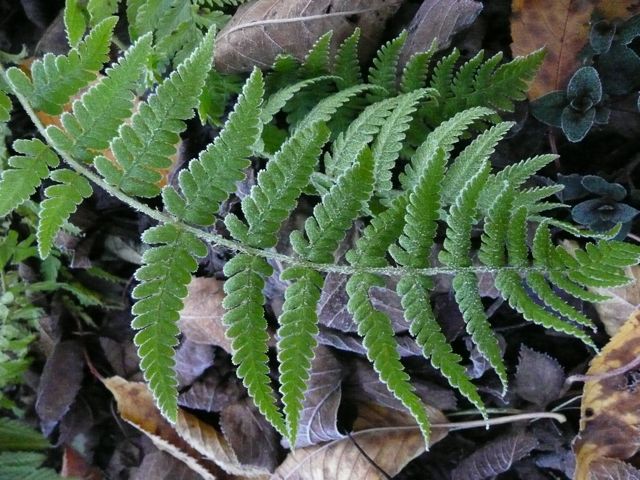This is a detailed top-down photograph taken outdoors featuring a green fern with 28 individual fronds. The fern's fronds resemble smaller, tree-like structures composed of tiny round leaves branching out from the main stem. The image also captures a surrounding environment with other plants, including smaller, rounded leaves similar to mint, particularly noticeable in the upper right quadrant where some have brown spots. The ground beneath the fern is scattered with brown, gray, and dark leaves, as well as some dark gray flowers and other natural debris, creating a textured backdrop of dry leaves, mold, compost, and organic remnants, all under natural light.